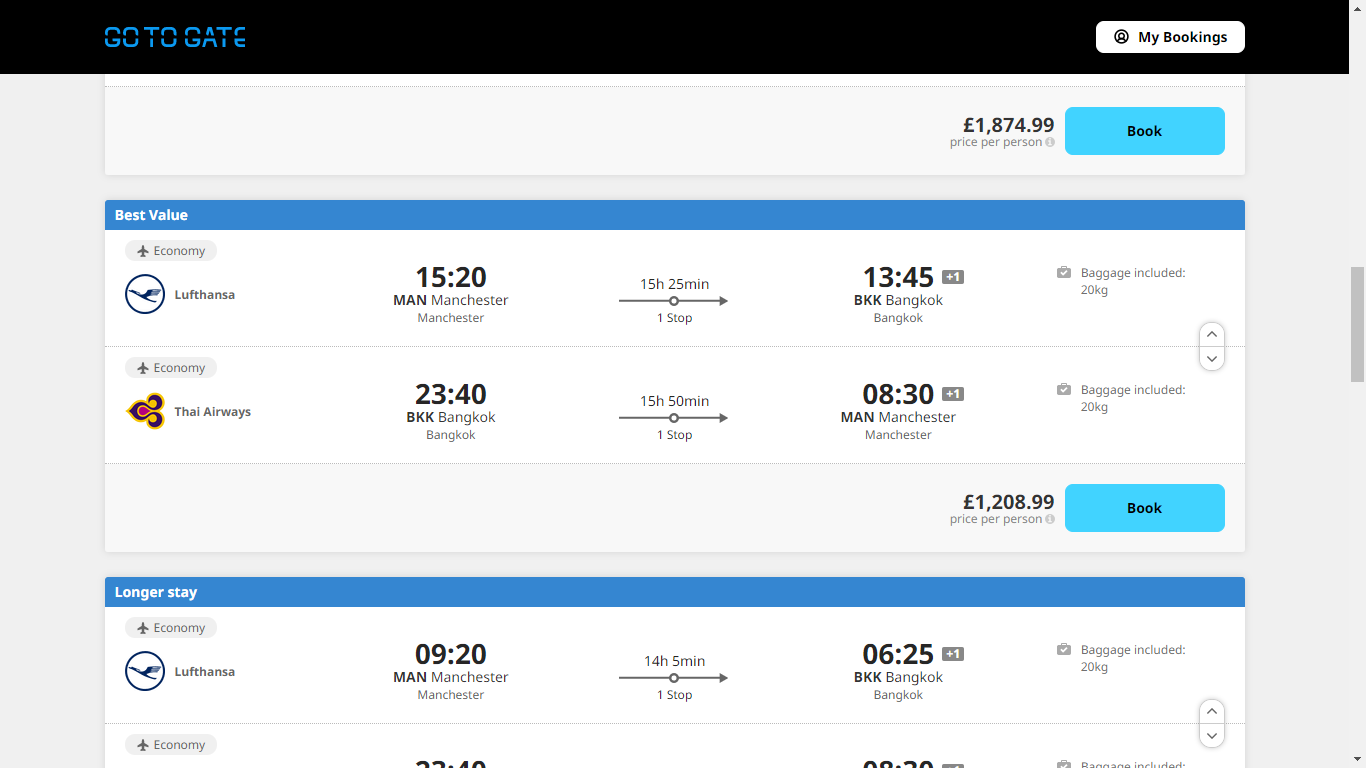At first glance, the page resembles a booking interface for airline tickets with a vibrant and clean design, dominated by bright colors and ample white space. At the top of the page, a prominent black banner captures attention. In the middle of this banner, deep blue, futuristic typography spells out "Go To Gate." Across from this, on the far right, a small but striking white box displays "My Bookings."

Below the banner, the layout is divided into two distinct sections, each marked by a bold and vivid blue line. The first section is labeled "Best Value," while the second section, at the bottom, is titled "Longer Stay." Both sections feature a selection of flights, complete with detailed information.

In the "Best Value" section, three flights are presented. The first flight is an economy option, indicated by the word "Economy" accompanied by a small airplane icon. Additionally, the airline logo for Lufthansa is displayed, characterized by its dark blue color and plane symbol. Each flight listing includes the flight path and times for departure and arrival. For example, the first flight departs from Manchester at 15:20 and arrives in Bangkok at 13:45 after a total flight duration of 15 hours and 25 minutes. The listing also specifies the number of stops.

The page continues to list two other flights, one featuring Thai Airways, recognizable by its distinctive yellow, red, and black logo. Information about included baggage allowances is provided for each flight, ensuring travelers are well-informed. The page also offers an option to book these flights directly, simplifying the booking process.